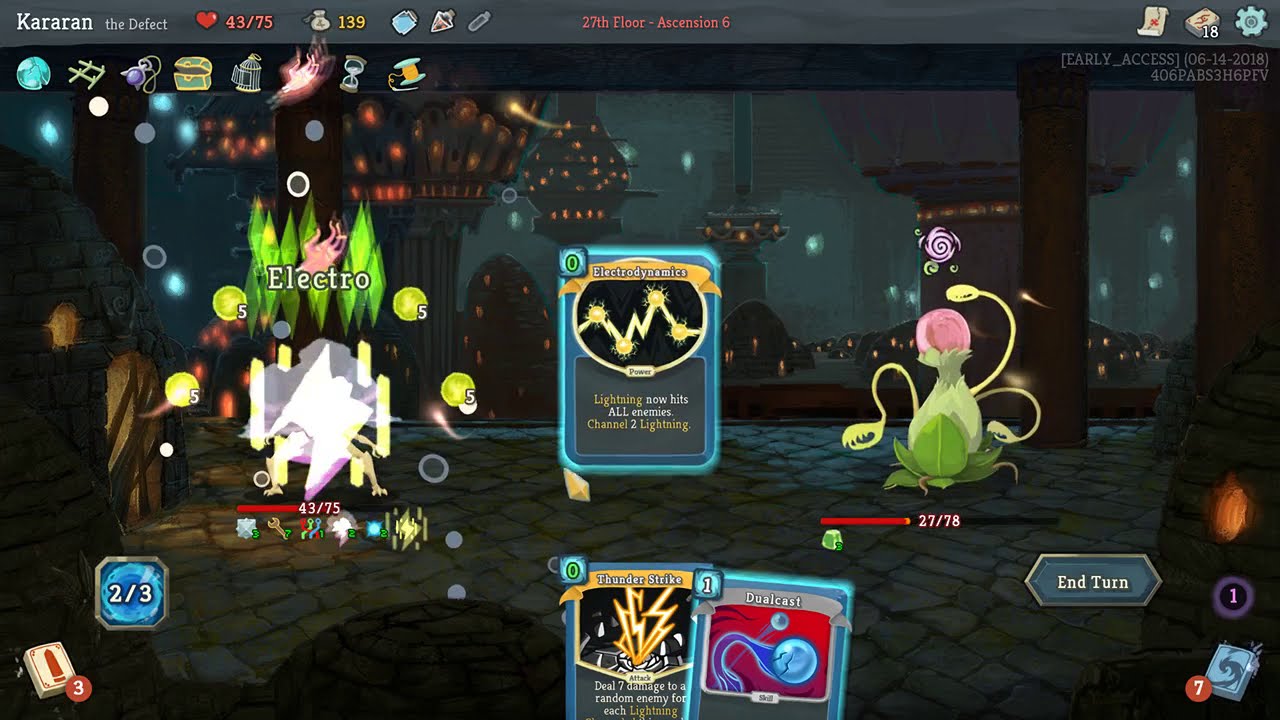This image is a detailed screenshot of a card-based video game featuring a turn-based battle scene likely set in a futuristic or fantasy setting. Dominating the screen is the game interface with a gray horizontal banner running across the top. From left to right, the banner reads "Kararon the Defect," highlighted by a heart icon with the stats "43/75" next to it, indicating the player's health. Beside these, a money bag icon shows "139," likely representing the player's gold or currency. Additional icons, including a jar of water, a spinning top, and a test tube, occupy the upper banner, hinting at various game resources or items. The top right corner of the banner displays three more icons, one of which appears to be a settings cog.

The main scene is set on a stone floor within a chamber featuring columned pillars that frame a large picture window, which appears to overlook either another room or an exterior scene, creating a sense of depth. On the right side of the screen, the word "Intern" is visible, possibly indicating the current game difficulty or player status. At the forefront of the scene are two uniquely shaped characters: the one on the right resembles a Venus flytrap-like plant, while the left character has an ambiguous, unusual shape. Each character has their life levels displayed below them.

Central to the gameplay, two cards are shown in the bottom middle section of the screen. One card is named "Electrodynamics" with the description, "Lightning now hits all enemies channeled to lightning." Below this, two additional cards are visible: "Thunderstrike" and "Dual Cast," indicating possible actions the player can take in their turn. Various other game elements, such as health bars and strategic icons, populate the bottom left and right corners, contributing to the overall complexity and engagement of the game's interface.